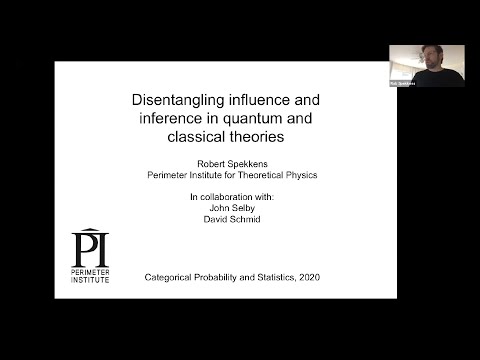The image features a screenshot of a computer screen with a picture-in-picture video chat. In the upper right corner, there's a man in a white room, wearing a dark shirt, identifiable by a name tag in the bottom left of his video frame. The main part of the screenshot displays a poster with a black border and a white background featuring black text. The text reads: "Disentangling Influence and Inference in Quantum and Classical Theories." Beneath the title, in smaller font, it credits Robert Speckens from the Perimeter Institute for Theoretical Physics, in collaboration with John Selby and David Schmid. At the bottom of the white section, it says "Categorical Probability and Statistics 2020." The bottom left corner features the logo "PI" and the text "Perimeter Institute."